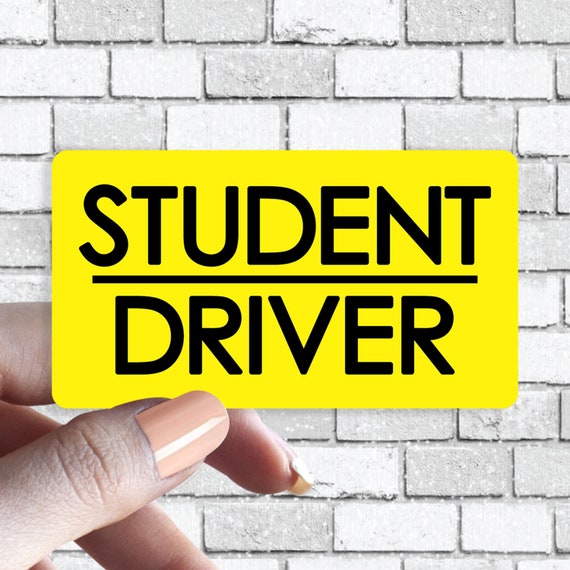In this square photograph, an elegant hand with tan or beige-painted nails holds a large, rectangular yellow card that reads "STUDENT DRIVER" in bold black letters. The hand, with fingers showing hints of a moderate brown or tan skin tone, is positioned in the lower left corner, gripping the card between the thumb, index, and middle finger. The card dominates the center of the image, standing out against the backdrop of a white brick wall. In the upper center part of the photo, there's a noticeable small crack in the brick, adding a touch of imperfection to the otherwise neat and tidy brickwork. This meticulously manicured photograph juxtaposes the vividness of the yellow card against the subtle tones of the wall, highlighting the message in a striking manner.